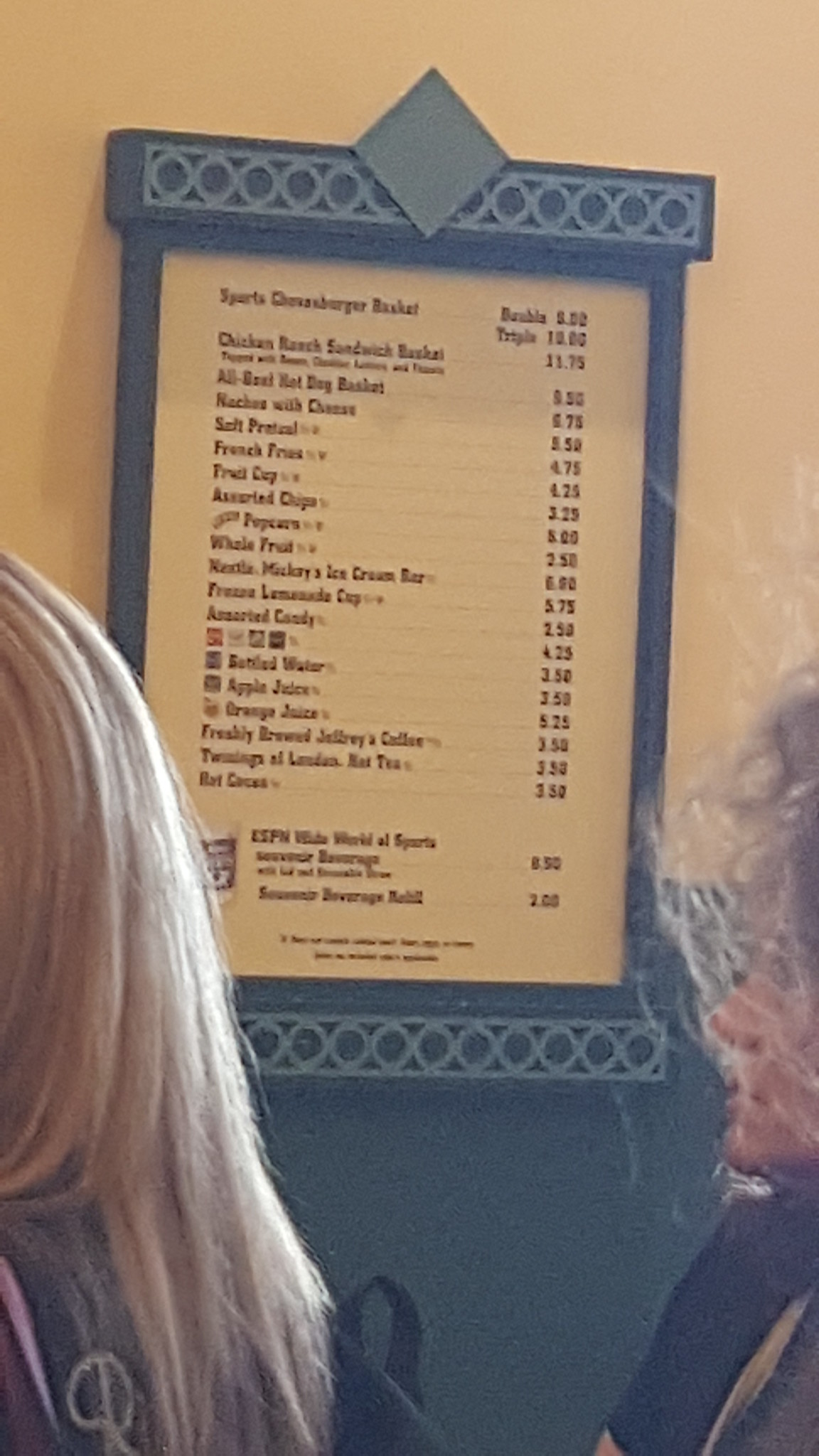Pinned to a wall, the image captures a blue menu board with intricate circular designs adorning the top and bottom. At the pinnacle of the board, a prominent diamond shape draws attention. The menu, fixed at a slightly tilted angle, features a beige interior card displaying the printed offerings, though the text is too small to discern without magnification. The beige of the menu blends seamlessly with the upper wall, exuding a "blue and dreamy" ambiance.

In the foreground, two individuals are engrossed in reading the menu. One, positioned with her back to the camera, has long blonde hair cascading down and is seen wearing a shoulder bag, indicated by the visible handle loop. The second person stands partially sideways, her disheveled hair partially obscuring her face. She is dressed in a navy front garment, layered beneath a slightly visible, khaki-colored overgarment. The scene merges detail with a touch of whimsy, providing an inviting yet mysterious glimpse into their moment.